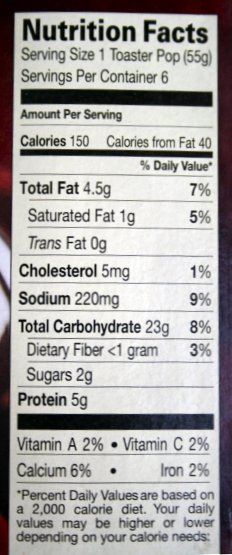This is a black and white nutrition label with a black border and various sections presented in the classic format. At the top, in large black bold letters, it says "Nutrition Facts." Directly below, in regular lettering, it states the serving size as one toaster pop (55 grams) and indicates there are 6 servings per container. A large black rectangular divider separates these details from the following information.

Underneath this divider, small bold lettering announces "Amount per serving," followed by another thin black divider. The label details that each serving contains 150 calories, with 40 of these calories coming from fat. 

A thicker black divider precedes the percent daily values section, marked by "Percent Daily Values" in bold black letters on the right side. The total fat content is 4.5 grams, accounting for 7% of the daily value, with saturated fat listed as 1 gram (5%) and trans fat as 0 grams. Cholesterol is at 5 milligrams (1%), sodium at 220 milligrams (9%), total carbohydrates at 23 grams (8%), dietary fiber less than 1 gram (3%), sugars at 2 grams, and protein at 5 grams.

At the bottom of the label, the vitamins and minerals are presented alongside small bold black dots. Vitamin A is listed at 2%, vitamin C at 2%, calcium at 6%, and iron at 2%. A concluding note mentions that these daily values are based on a 2,000 calorie diet, with the caveat that individual daily values may be higher or lower depending on specific calorie needs.